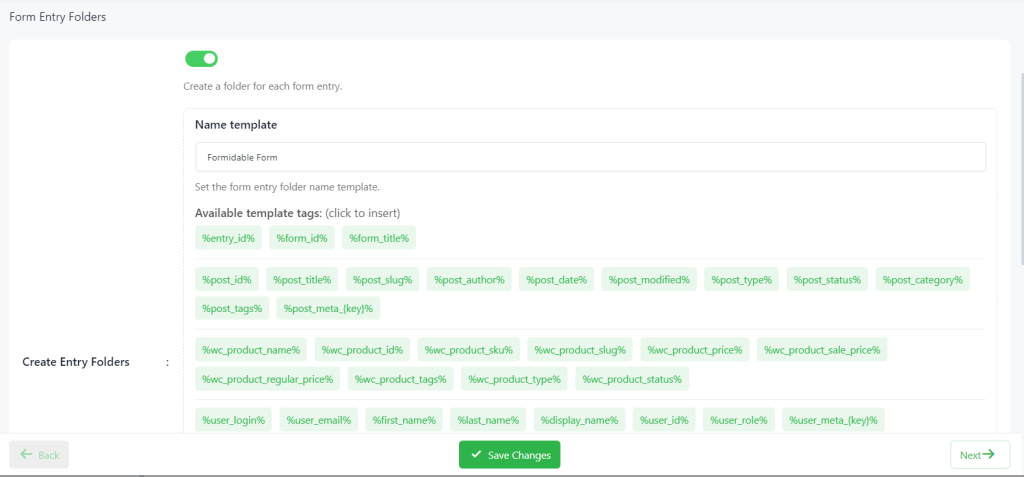This image captures a webpage displayed on a computer screen. At the top of the page, there is a gray bar with the text "Form Entry Folders" written in black. Below this gray bar, the background is white. Approximately one and a half inches to the right of the gray bar, there is a green radio button with a white circle. This button appears to be in the "on" position. 

Directly below the gray bar is the instruction "Create a folder for each form entry." Below this, the text "Name Template" is prominently displayed in bold. Underneath the bold text, "Formidable Form" is written in regular text. Further down, there's a note stating "Set the form entry folder name template."

Beneath this note is a darker print that reads "Available Template Tags - Click to Insert." Below this text, there are multiple rows of light green tags with dark green print, though the tags’ text is difficult to decipher. The first row contains three tags, the second row has nine tags, the third row holds two tags, the fourth row includes six tags, the fifth row has four tags, and the sixth row features eight tags. Each row is comprised of these template tags, which are intended for insertion into form entry folder names.

At the very bottom of the page, centrally located, there is a dark green button with a checkmark icon and the words "Save Changes" written on it.